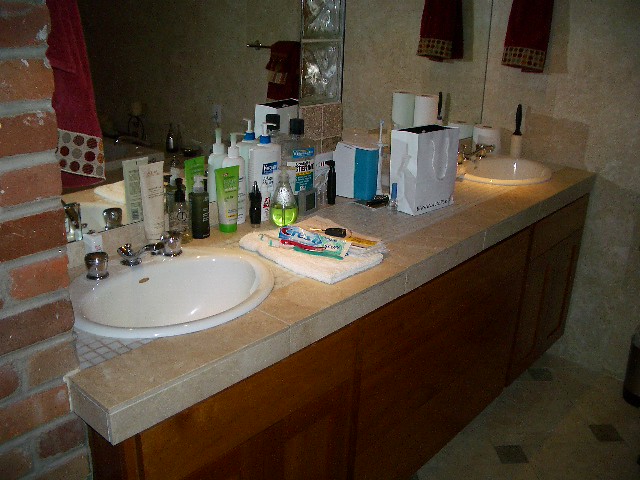The image displays a well-appointed bathroom with a sophisticated design. Dominating the scene is a beige stone countertop with pristine, straight edges. To the left, a striking brick wall comprised of reddish bricks and mortar lends a rustic touch to the setting. Beneath the countertop, medium-brown wooden paneling provides a warm, natural contrast.

The flooring is adorned with marble-like tiles that extend partially up the opposite wall, enhancing the bathroom's elegant aesthetic. Behind the countertop, a mirror reflects a bathtub in the background, partially concealed by a red shower curtain featuring a white stripe and a playful pattern of multicolored circles.

On the lefthand side of the countertop sits a white basin sink outfitted with sleek silver faucets and handles, mirrored on the right-hand side. The central area of the countertop is cluttered with personal items, including a white bag, a white towel topped with Crest toothpaste, and an array of skincare and lotion products. Among the assortment of roughly 20 bottles are a white bottle with a blue cap, a green bottle with a green cap, and a Listerine bottle with a black cap. These items are scattered across the countertop, adding a touch of realism to the scene.